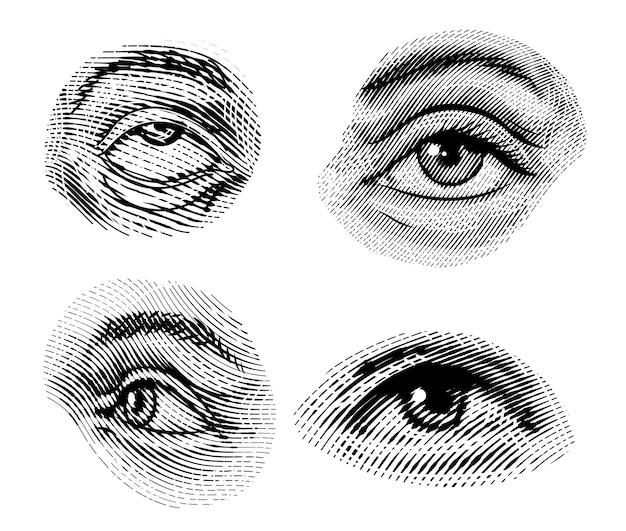This black and white square-shaped image features four distinct line drawings of human eyes, arranged in a 2x2 grid with a white border both behind and around each eye to keep them separate. The eyes appear male-like, depicting various gazes and expressions. 

- The top left illustration shows a right eye looking upwards with a thin black eyebrow and thin black and white lines running through the image, exposing the white area extensively under the iris.
- The top right image portrays a left eye looking straight ahead. It has a thin black eyebrow and thicker upper eyelashes, with intricate thin black lines across the illustration.
- The bottom left eye, which has a slightly thicker eyebrow than the others, is looking to the left, exposing the white side of the eye to the viewer.
- The bottom right showcases another right eye, this one gazing towards the top right corner. It has an enlarged pupil and a vaguely visible thin eyebrow, with a darker patch at the top of the iris.

Each eye illustration maintains a slightly distorted circular shape and is rendered with a distinct line contour filter, emphasizing the differences while keeping a stylistic cohesion. The eyes appear to belong to different individuals, providing a diverse range of expressions within the artwork.